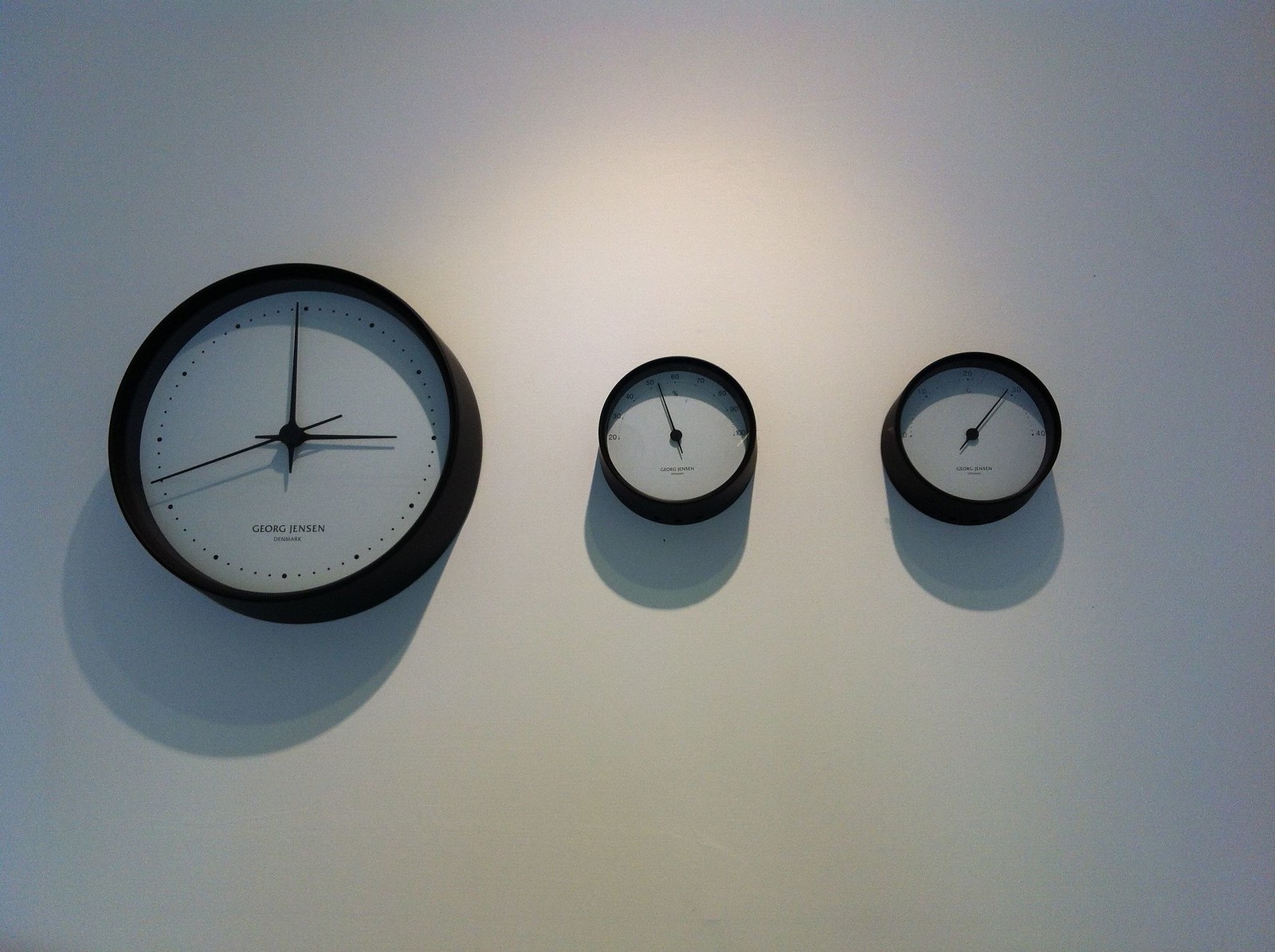In this image, a round clock is mounted on a pristine white wall. The clock's housing is sleek and black, contrasting against its white face. Instead of traditional numbers, the clock features minimalist dots marking the hours. The black clock hands stand out sharply against the white background, making them easy to read. Adjacent to the clock, there is a thermometer or temperature gauge, visually similar to the clock with a white face, black numbers, and a black hand. To the far right, there is another instrument, likely a humidity gauge, although its details are not entirely clear. It follows the same design language as the clock and thermometer, with a white face, black numbers, and a black hand. The clock bears the inscription "Georg Jensen, Denmark," indicating the prestigious Danish manufacturer responsible for these stylish and functional timekeeping and measurement devices.